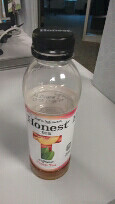The image depicts a bottle of Honest Tea, specifically a peach-flavored variety, situated on a tabletop within a domestic environment. The bottle is more than halfway empty and features a black cap. A white label adorned with illustrations of peaches and a tea leaf encircles the bottle, prominently displaying the "Honest Tea" brand name. The scene captures a candid snapshot, likely taken with a phone, and shows a partial view of the kitchen and adjacent room in the background, including sections of the floor and door. The bottle is angled slightly downwards, clearly showcasing its contents.